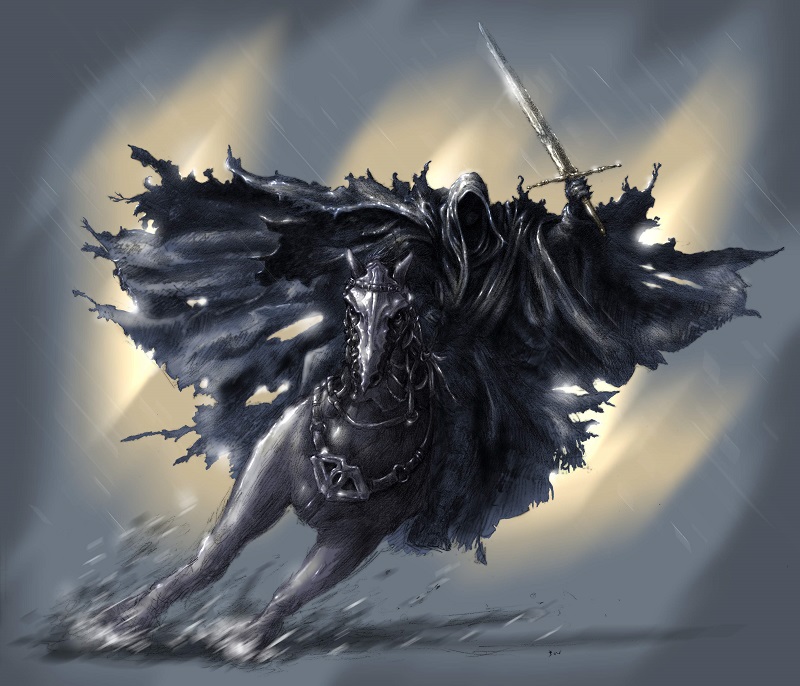In this striking illustration, a hooded and mysterious figure rides a dark horse, charging directly towards the viewer. The background features a dramatic interplay of grays, light blues, and whites, resembling a gray curtain with light shining from behind. Despite the overall gloominess, a subtle yellow light effect adds depth to the scene, giving the impression of rain falling and creating a dynamic atmosphere.

At the forefront, the dark, almost spectral figure is draped in a tattered cloak that extends outward like jagged wings, complete with holes that let the background light shine through. Though the interior of the hood is shrouded in darkness, perhaps hinting at a faint chin, the face remains mostly obscured. 

Riding a horse that appears to be leaning sharply to the left, as if sliding through mud or making a swift turn, the figure’s menacing presence is accentuated by the horse’s metal headpiece and reins, which drape elegantly over its shoulders and under its body. The horse's facial detail is intricate, with metallic elements adding to its imposing appearance.

The rider's left arm is raised, gripping a large, gold-handled sword. This weapon gleams menacingly, with a noticeable glimmer halfway down its length, its tip reaching skyward. The figure’s hand, encased in what appears to be a metal glove, firmly holds the sword, signifying readiness and power. This artwork captures an intense, almost haunting moment, steeped in dark, evocative detail.